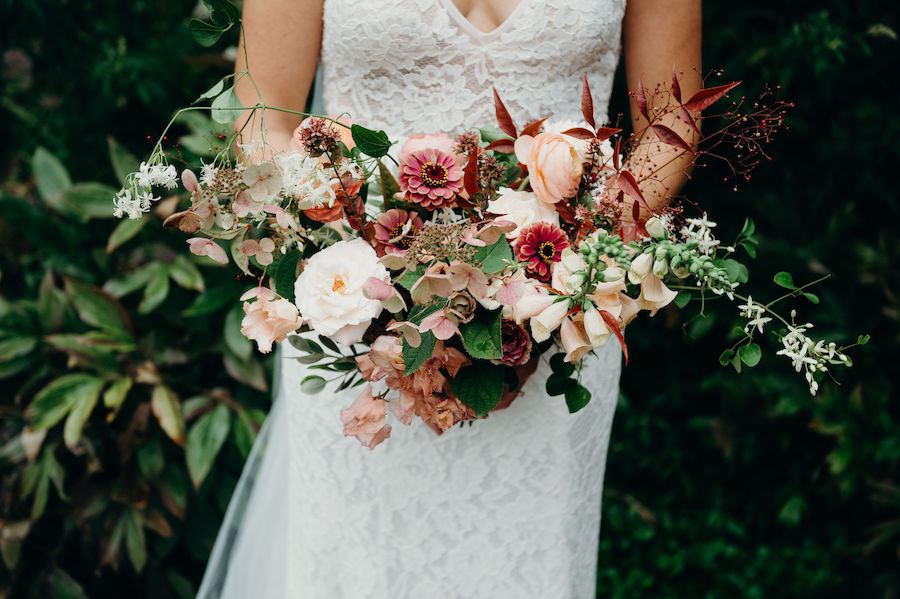In this professional portrait taken in daylight, a bride is prominently featured at the center of the image, facing the camera. She is adorned in a sleeveless, white wedding dress that is low cut, revealing a bit of her cleavage. The photograph captures her from the chest down, without showing her face or shoes. The bride holds a large bouquet that obscures her hands; the bouquet is comprised of various flowers in shades of light and dark pink, along with white blossoms, and accented by green leaves. The background is filled with lush green plants and bushes, further emphasizing the natural and serene setting of the shot. No text is present on the image.